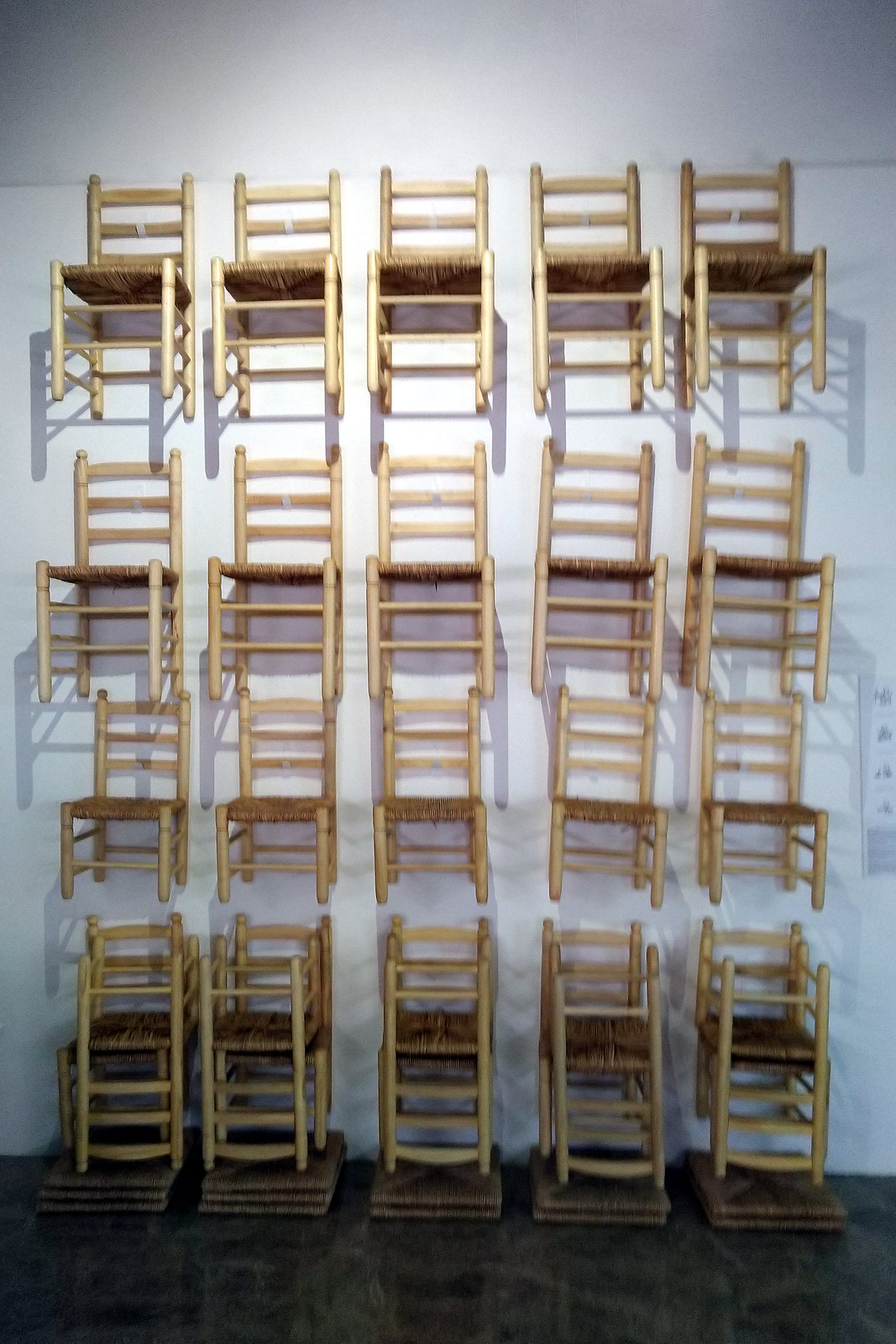In this surreal photograph, we see a plain white wall in the background adorned with a unique arrangement of wooden chairs. The chairs, which appear to have wicker or straw seats and simple backrests with three slats, are arranged in four rows of five. The bottom row of chairs is placed on dark, possibly carpeted tiles, featuring a peculiar setup where two chairs are stacked against each other, one right side up and the other upside down, making their seats touch. The three rows above them seem to be hovering, creating an illusion of floating chairs, though it isn’t clear how they are affixed to the wall. The floor is a dark gray to almost black color, contrasting starkly with the lighter wall. This arrangement might be an art piece or a means of displaying the chairs for sale, possibly for a restaurant setup. Shadows cast by a light source above add to the mystery and visual intrigue of the display.